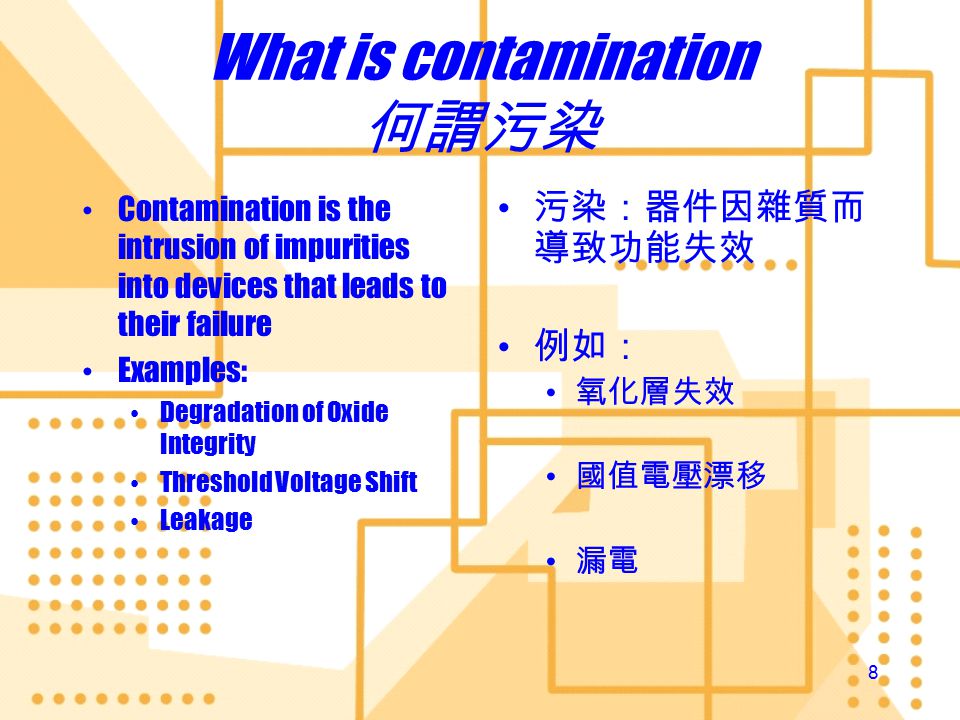The image is a detailed slide from a PowerPoint presentation, used as an advertisement or notice, with a white background adorned with light decorative elements, including brown and orange lines, dots, and triangles—all intersecting to form a complex pattern. At the top of the slide, bold blue lettering poses the question "What is contamination?" accompanied by Korean characters. On the left side, a bulleted list in English explains that "contamination is the intrusion of impurities into devices that leads to their failure," providing examples like the degradation of oxide integrity, threshold voltage shift, and leakage. Mirroring this layout, the right side similarly features Korean text structured with bullet points, effectively translating the same information. The dots and lines add to the aesthetic, with yellow dots forming a square grid on one side, enhancing the overall visual design of the slide.